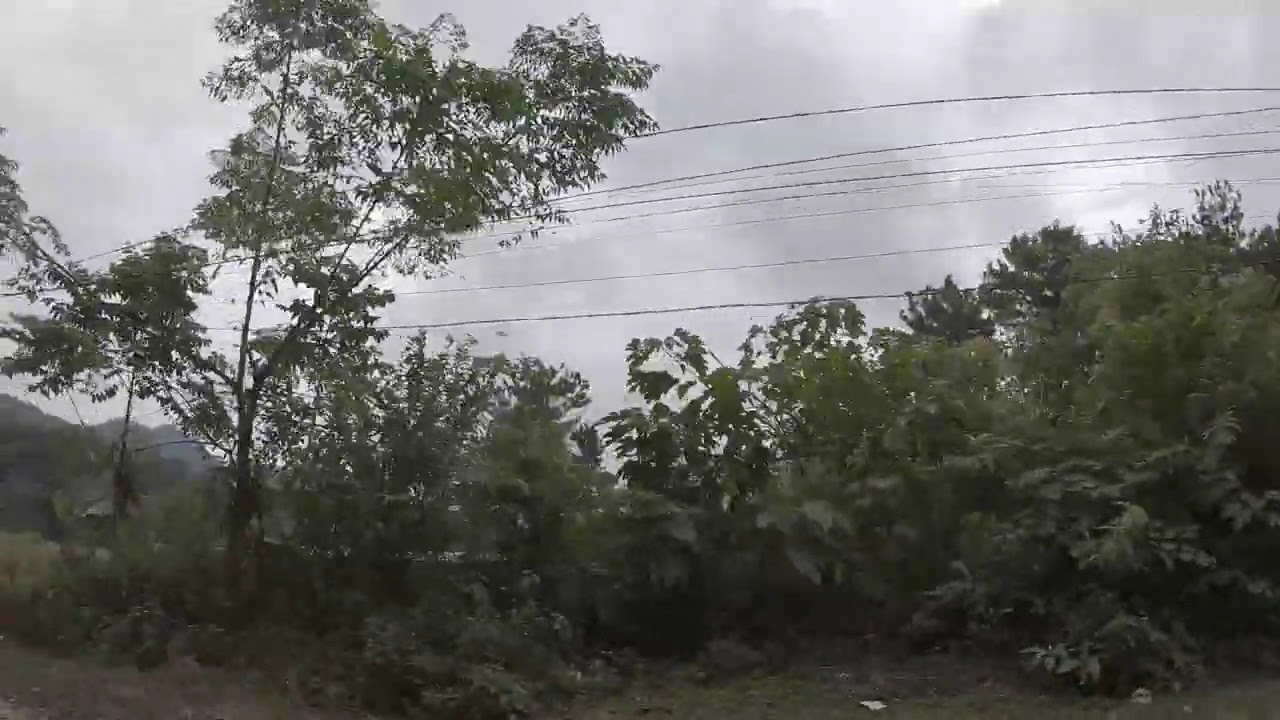This color photograph, taken in a grainy, low-quality style reminiscent of a still from a video, captures a landscape in a tropical or subtropical setting. The image, oriented in landscape format, features a prominent, tall, skinny tree on the left and an assortment of smaller bushes and medium tall trees spread across the right side. A small clearing appears in the foreground. Overhead, approximately eight or nine power lines stretch across the entire width of the photo, from left to right, intersecting with the tops of the shorter trees and passing behind the taller tree. The gray, cloudy sky dominates the background, giving the weather an overcast, almost smoky appearance, with no hint of blue visible. Behind the row of trees, hints of a distant landscape, possibly featuring gray hills, can be discerned on the horizon, adding depth to the scene. The photo, void of any text or people, adheres to a photographic representational realism style.